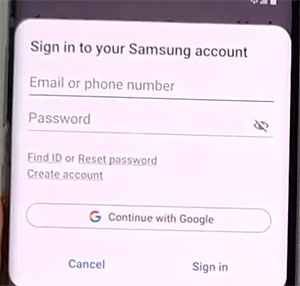The image depicts a login page for a Samsung account, prominently displayed on what appears to be a smartphone screen. 

At the top of the page, there is a horizontal black bar. Below that, on a stark white background, is the heading "Sign in to your Samsung Account" in black text. 

The login form begins with fields for "Email or phone number" followed by "Password," which includes a button to reveal the entered password. 

Lower on the page, there are options to "Find ID or reset password" and "Create account" for users who need assistance or wish to register.

Adjacent to these options, a button labeled "Continue with Google" appears, featuring Google's multicolored logo in red, yellow, green, and blue.

At the bottom of the page, two prominent blue buttons are placed: "Cancel" and "Sign In." 

The overall design of the page is simple and functional, focusing on usability with predominantly black text and a few colorful elements for interactive options.